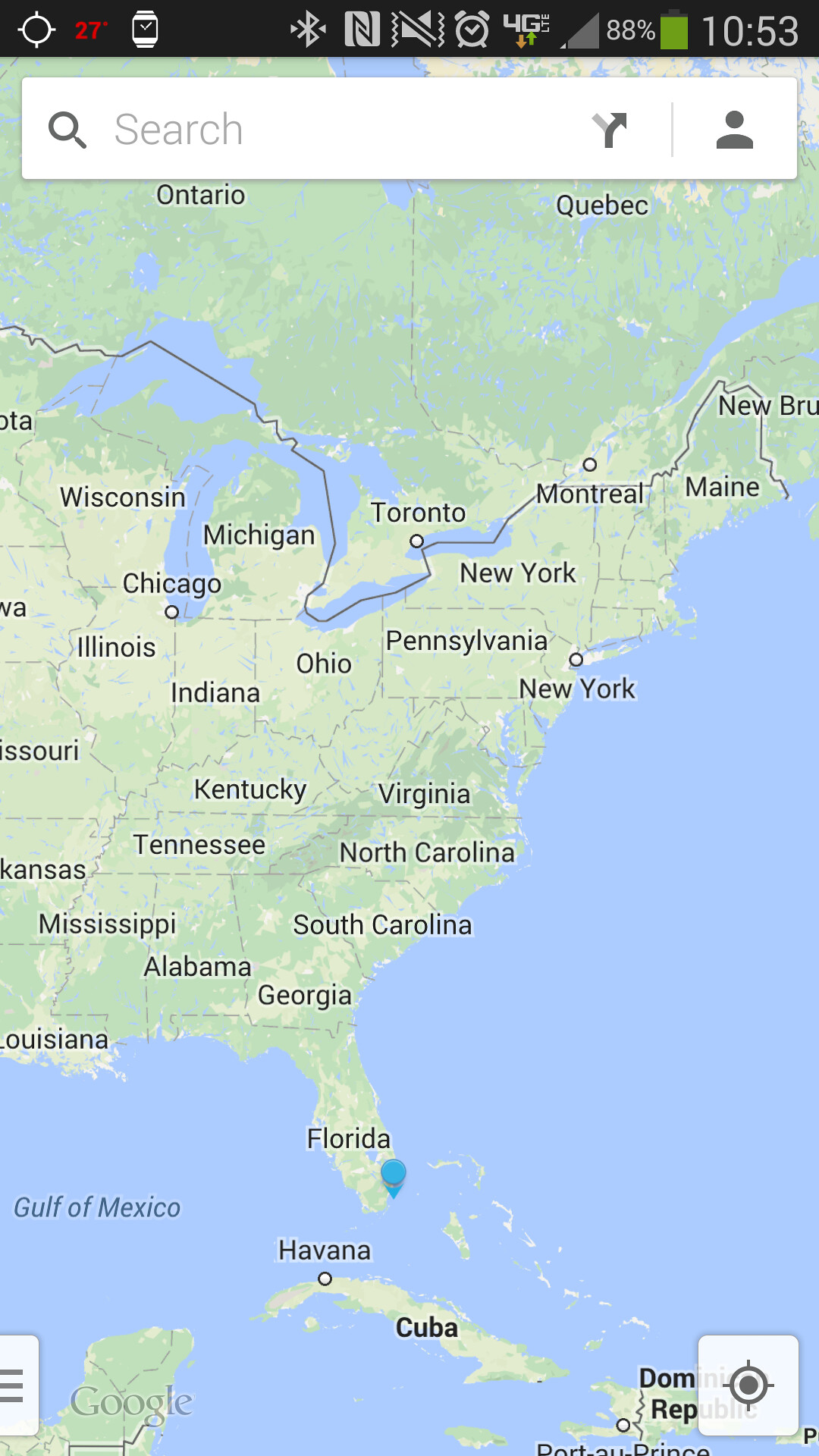A detailed screenshot from Google Maps displayed on a smartphone shows a geographical span from Ontario and Quebec in Canada through the eastern United States down to Central America, including Haiti, the Dominican Republic, and parts of the Gulf of Mexico. The top of the image features a black status bar, indicating various phone statuses: a red 27-degree temperature symbol, a clock face icon, the Bluetooth symbol, and an icon indicating vibration mode. Additional icons display a set alarm, 4G LTE connectivity with minimal signal strength (one grey bar), an 88% battery level, and the current time as 10:53. Underneath the black bar is a white search bar accompanied by a grey right-turning arrow and an icon of a person. The map specifically highlights U.S. states from Wisconsin down to Florida on the eastern side, extending west to Illinois, Missouri, Arkansas, Mississippi, and Louisiana. Notable cities and regions such as Chicago, Maine, New Brunswick, and New York are visible. The user's location is pinpointed near the bottom of Florida, and surrounding water bodies like the Gulf of Mexico and the Atlantic Ocean are represented in blue.